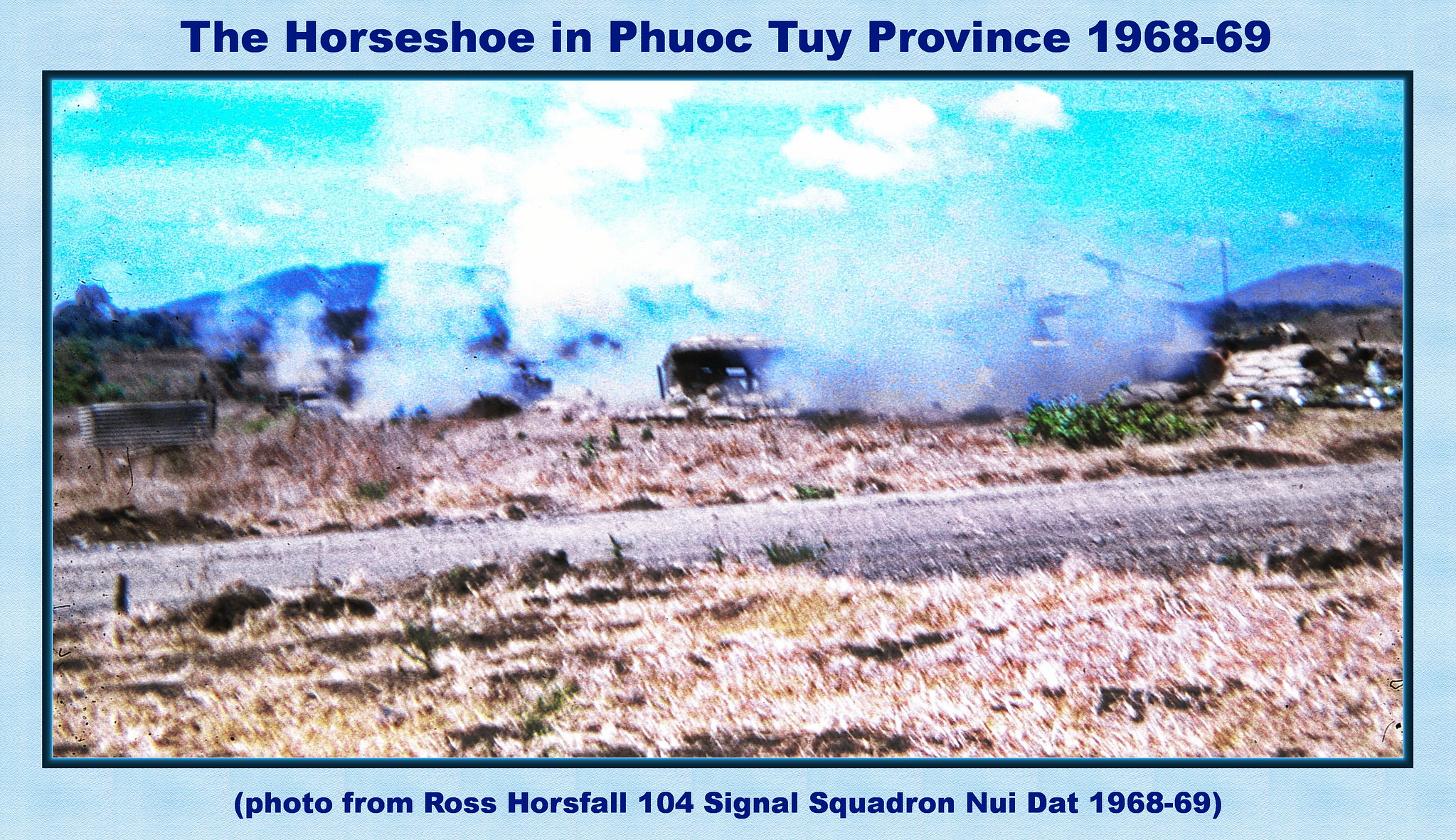This postcard-style image, titled "The Horseshoe in Phuoc Tuy Province, 1968-69," captures an outdoor scene filled with wartime elements. The photograph, outlined by a thin dark blue border, was taken by Ross Horsefall of the 104 Signal Squadron, Nui Dat during 1968-69. The sky is a striking turquoise blue, cluttered with clouds or possibly white smoke. At the forefront, the ground is a spread of brown, dead grass or weeds. A narrow gravel road runs horizontally through the middle of the image. On the opposite side of the road, the ground appears to be smoldering, with white smoke rising near a central, black, square object. Towards the right of the smoke, a hint of green shrub emerges. The background reveals distant mountains and random green trees, giving a sense of depth to this vivid yet hazy scene. The overall setting suggests a deserted field or an abandoned area under the broad daylight, encapsulating the harsh and chaotic environment of Phuoc Tuy Province during the mentioned period.